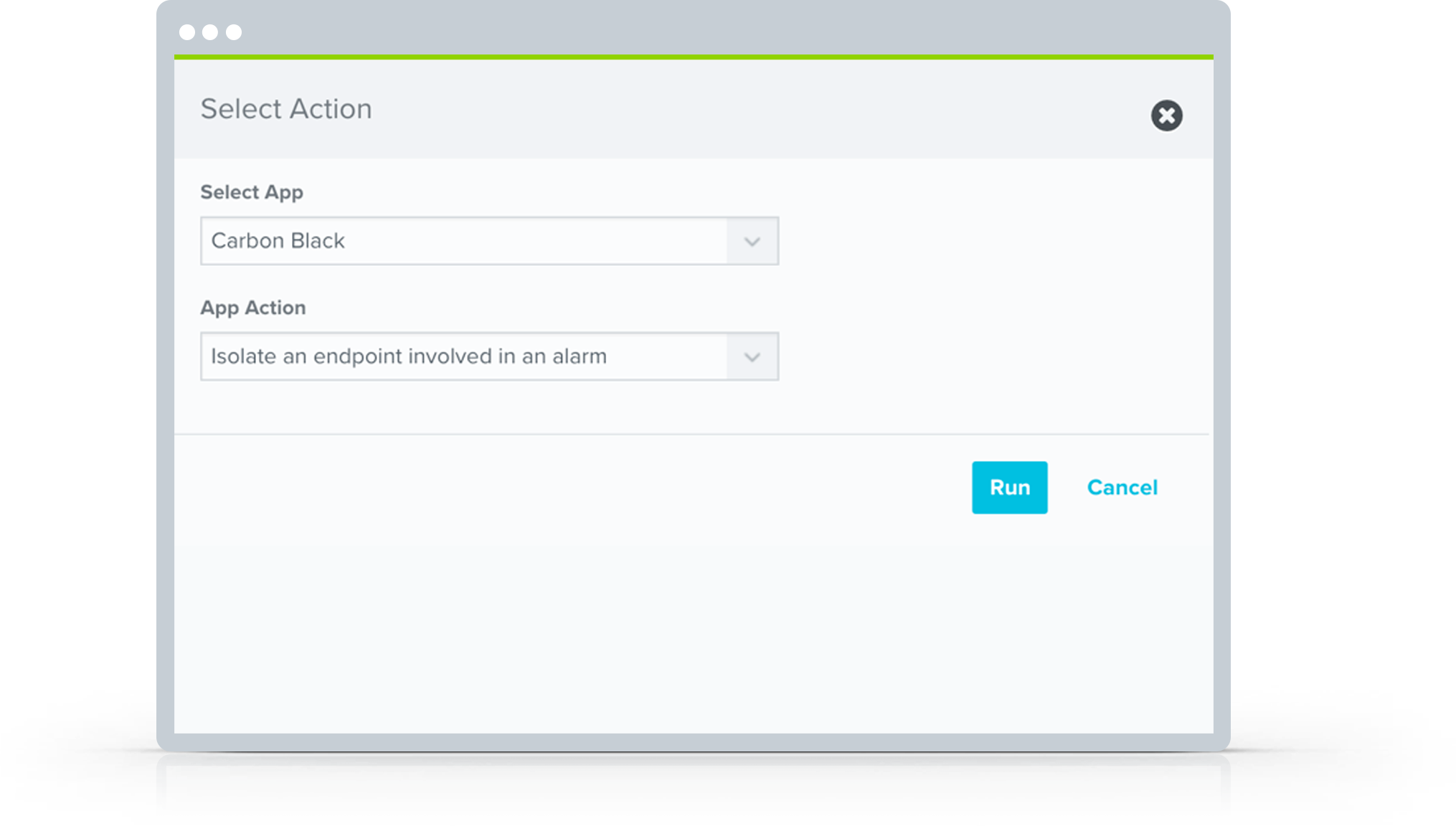A detailed cropped screenshot of a large "Select Action" dialog box is presented against a muted grey background, accented by three horizontal dots at the top center. Below the dots are a series of white dots, and beneath those, a thin grey horizontal line spans the width of the dialog box. The top left corner of the box prominently displays the text "Select Action". On the top right corner, there is a circular black button with a white 'X' in the center, serving as a close button.

Directly under "Select Action", on the left side, the label "Select App" is clearly visible. A drop-down box immediately follows where "Carbon Black" is selected. Further down, the text "App Action" introduces another drop-down box, which has "Isolate an Endpoint Involved in an Alarm" chosen from its options.

Towards the lower right section of the dialog box, a vibrant blue button inscribed with "Run" is placed, signaling an actionable command. Adjacent to the "Run" button, to the right, is a "Cancel" option written in standard blue font without a surrounding box. The overall interface elements are clear and neatly organized within the dialog box on the light grey background, denoting a well-structured software interaction window.